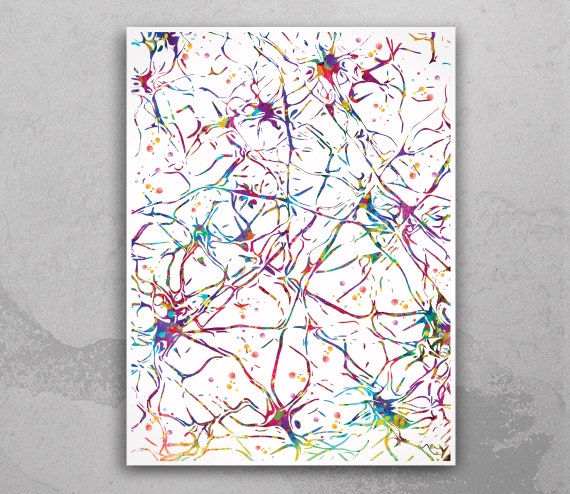The image depicts an abstract painting set against a gray wall that features subtle dark gray streaks. The artwork itself is on a white rectangular canvas and is composed of intricate, blood vessel or neuron-like designs with wiry, tentacle-esque lines extending from diamond-shaped central bodies. These lines are rendered in an array of vibrant colors, including red, green, blue, purple, pink, orange, and dark purple, creating a rainbow effect. The overall effect is reminiscent of neural connections or an electric network, with the colorful lines scattered across the entire white canvas, providing a sharp contrast to the subdued background.